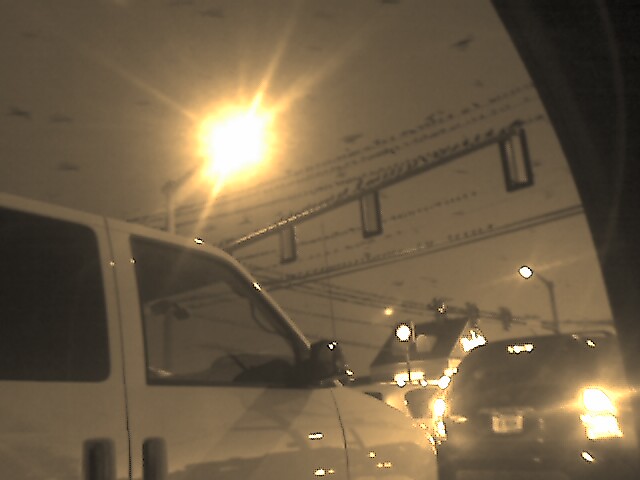The image depicts a group of cars stopped at a traffic light, with a particular focus on a dark-colored car with its brake lights illuminated directly in front of a white van, which has a sliding door featuring a dark window and a clearer window on the passenger side. The scene is likely taken from inside another vehicle, suggested by the partial view of a window frame on the right side. Overhead, a network of electrical wires is heavily populated with birds, creating a striking contrast against the sky. Despite the overall shadowy appearance, sunlight is visible, hinting that the image might have been captured through a tinted window. The background features various streetlights and traffic signals, with one particularly bright streetlight shining down, which contributes to the unusual lighting and somewhat surreal atmosphere of the scene. The composition gives the impression of a busy, yet somewhat ambiguous urban environment, blending realistic vehicular details with a strangely abstract background.